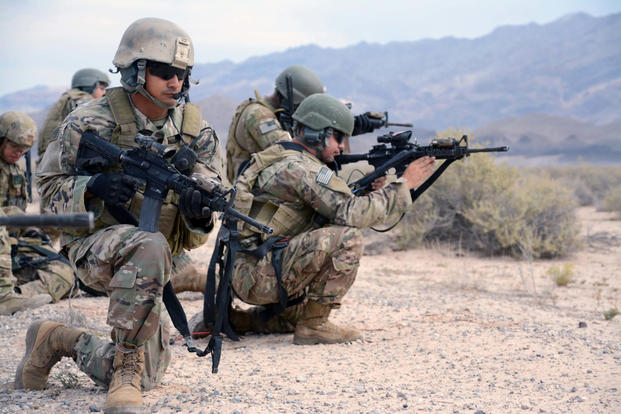In this detailed, up-close photograph, several U.S. soldiers are depicted in a combat position, each crouched down on one knee and holding tactical assault rifles. The soldier in the bottom left-hand corner wears sunglasses along with a complete set of combat gear: helmet, jacket, pants, boots, and a carbon stock rifle with a black, gunmetal finish. To his right, two more soldiers are seen in scope mode, aiming their rifles across a large valley that stretches out behind them, framed by mountainous hills. Amongst the arid, reddish-tinted, dry sand terrain, sporadic green bush-like plants can be seen. The overall scene is set against a backdrop of mountains tinged with shades of brown and green under a gray sky. Most soldiers are equipped with goggles, backpacks, and vests, and one soldier has a headset. Their army fatigues indicate a U.S. Air Force origin, supported by visible American flag patches on their uniforms. The image captures a sense of readiness and tension, whether it portrays an actual war scene or a military training exercise.